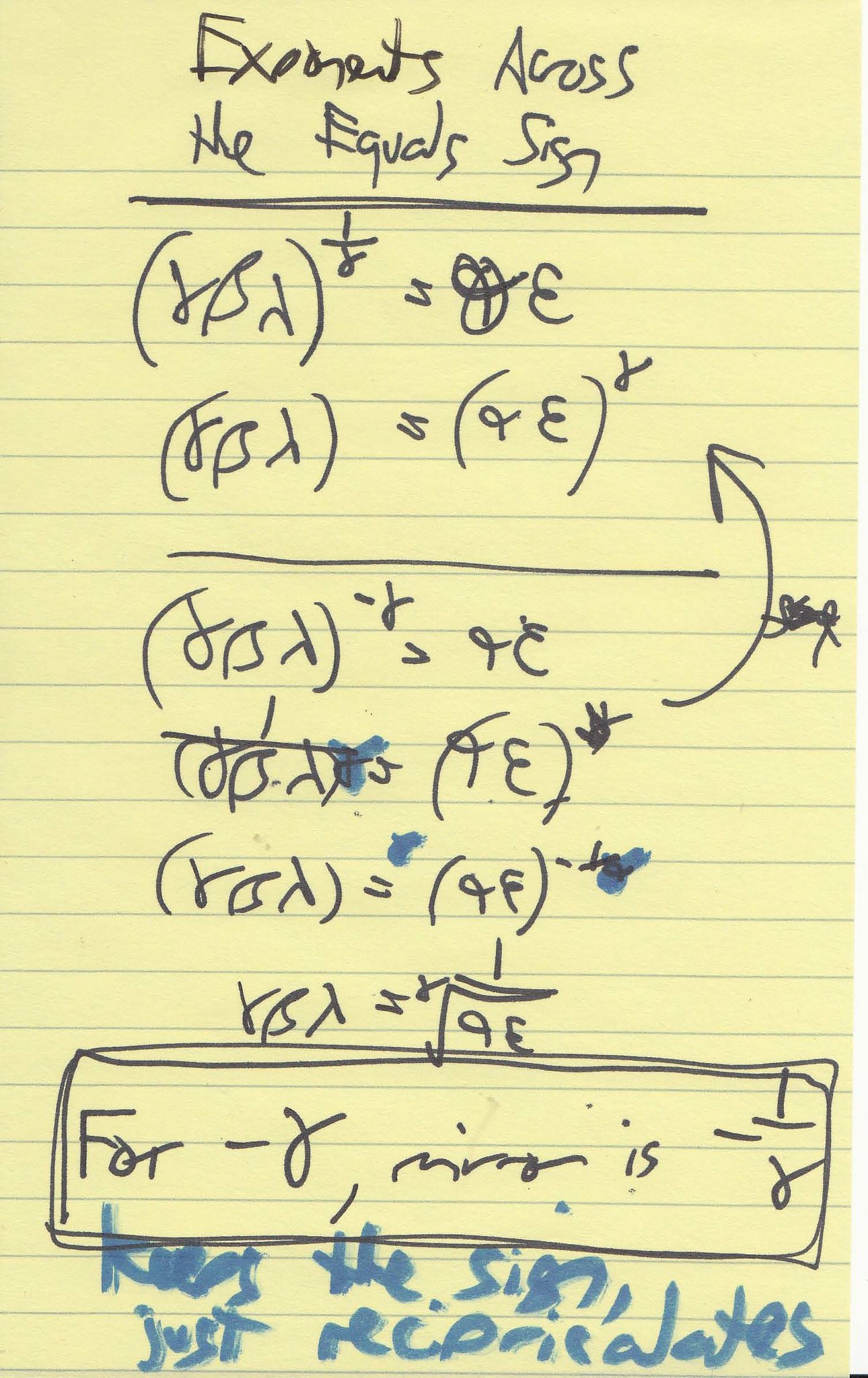This is an image of a rectangular sheet of yellow notebook paper featuring a series of handwritten mathematical expressions. Horizontal lines run across the paper, typical of notebook pages. 

The majority of the writing appears to be done in black ink, presumably from an ink pen. At the top of the page, in particularly messy handwriting, are the words "Exponents Across the Equal Sign," indicating the likely subject of the notes.

The page contains multiple mathematical equations, characterized by the use of parentheses, equal signs, greater than signs, and other mathematical symbols. These equations are aligned vertically, with at least six or seven distinct expressions filling the page. Additionally, there are a couple of thick horizontal lines separating sections of the page.

Toward the bottom of the paper, there is a note written in blue marker that reads "Keep the sign just reciprocates," though its meaning is unclear. The blue marker is also used to highlight or star certain parts of the black ink writing, intersecting with some of the equations and annotations, adding to the overall messiness of the presentation.

Overall, this image captures a somewhat chaotic and hurried attempt at documenting mathematical concepts, with the use of different colors and the sloppiness of the handwriting contributing to its haphazard appearance.